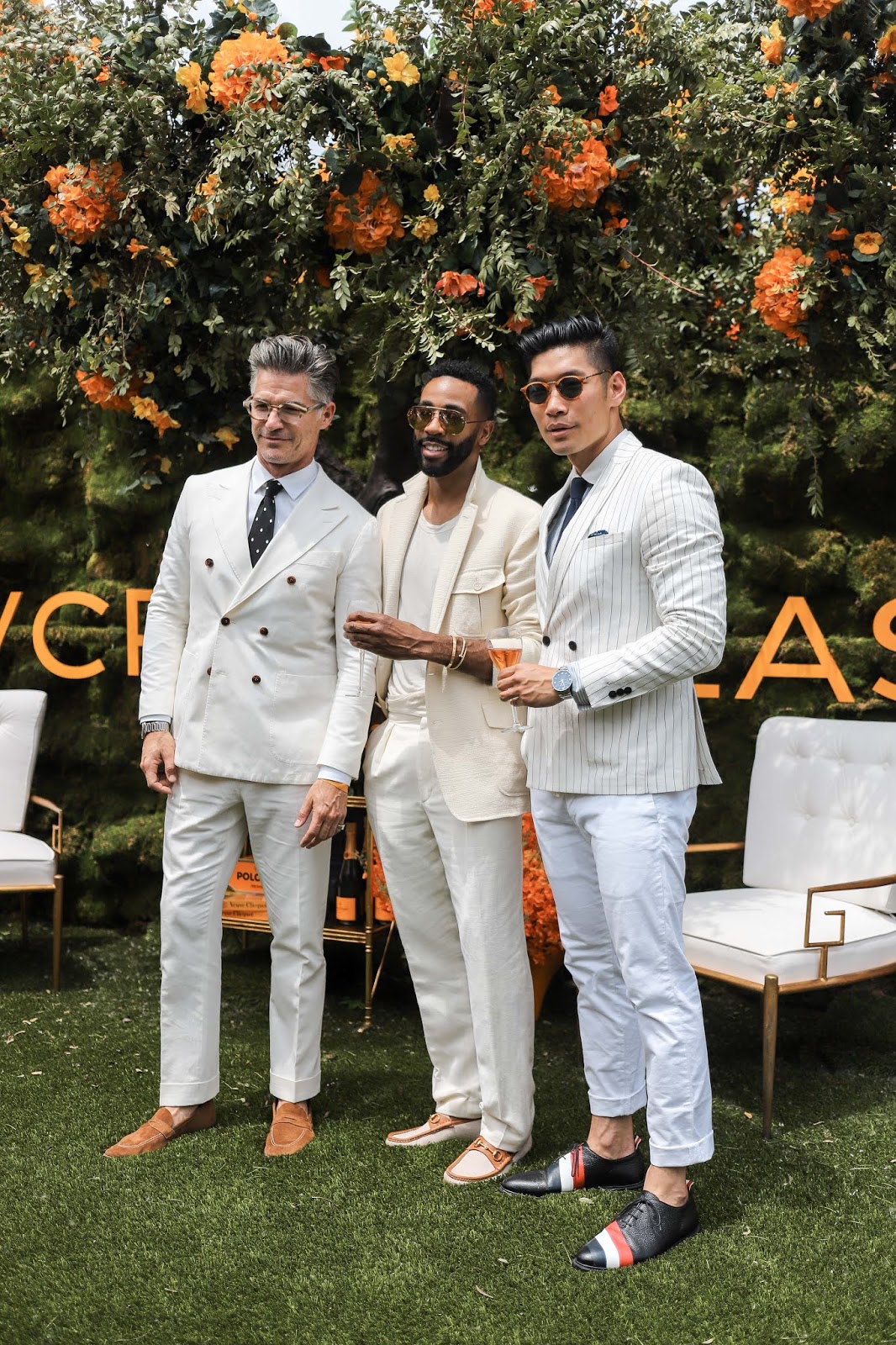This photograph depicts three well-dressed men standing closely together on a grassy lawn, framed by a vibrant floral and greenery backdrop that features trees with pink and orange blossoms. The trio includes a white man on the left, tinted glasses perched on his nose, a black man in the center wearing sleek sunglasses, and an East Asian man on the right, also sporting sunglasses. Each is adorned in stylish summer suits in shades of white and beige; the white man completes his look with suede brown loafers, the black man with white and tan loafers, and the Asian man with black shoes featuring a distinctive red and white stripe across the toe, without socks. Two chairs, one white and one orange, flank the men. Behind them, partially obscured lettering—potentially forming the characters C, P, A, and S—further decorates the backdrop, matching the color scheme of the surrounding flowers. The men hold cocktails and gaze off to the left, seemingly poised for another picture, while someone captured this candid moment.